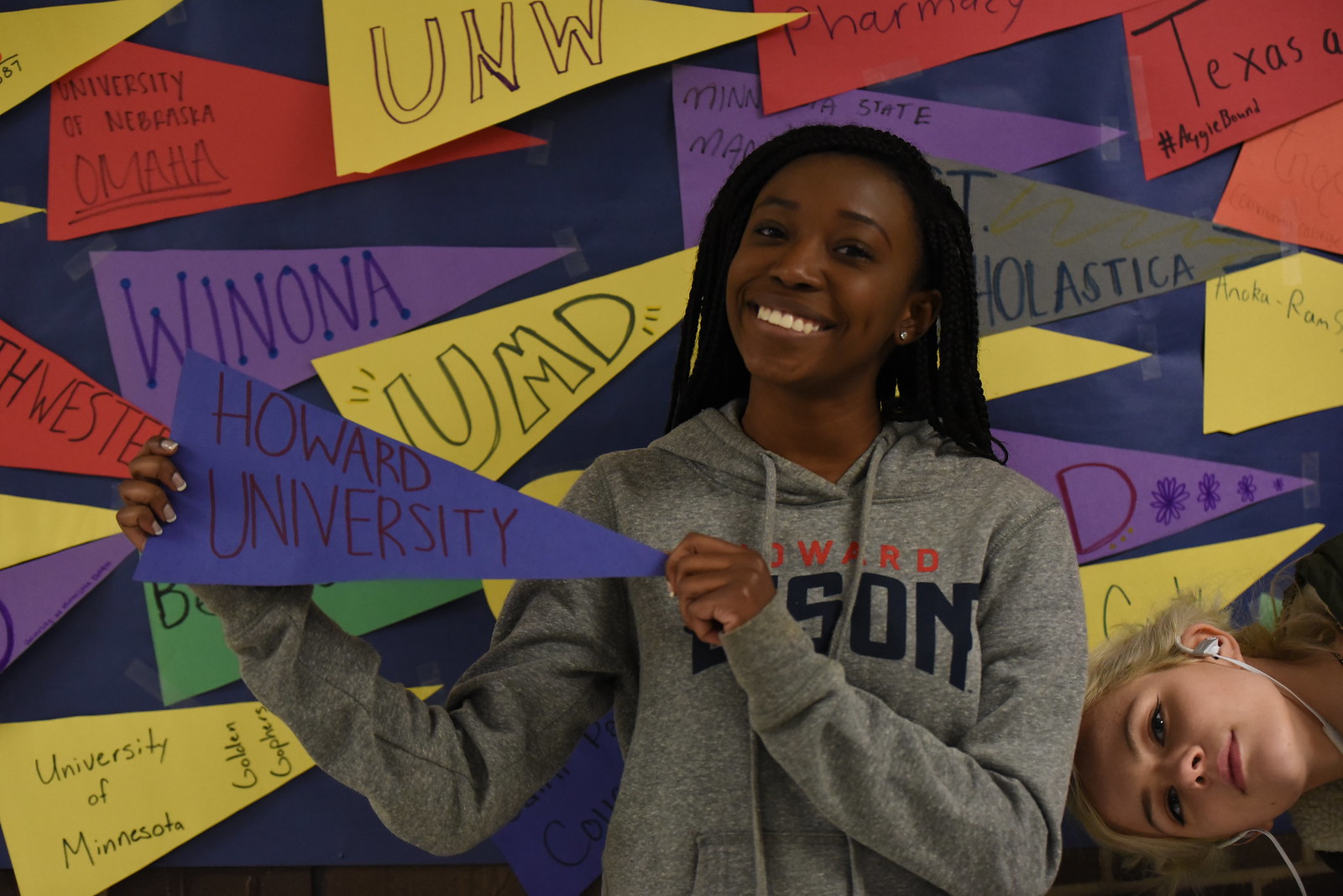In this vibrant indoor photograph set in a high school, two girls are the focal point. The black girl stands proudly at the center, her broad smile lighting up the room. She wears a gray hoodie and holds a blue triangular pennant reading "Howard University" in white letters. Around her, pinned to the wall, are similar pennants with names of various universities, signaling a celebratory college acceptance event. To her right, in the bottom right corner of the image, a blonde Caucasian girl is lying down with her head tilted sideways. She has headphones in her ears, as if she's listening to music, and looks directly at the camera. The joyful atmosphere and the array of colorful college pennants suggest a milestone moment for these students.